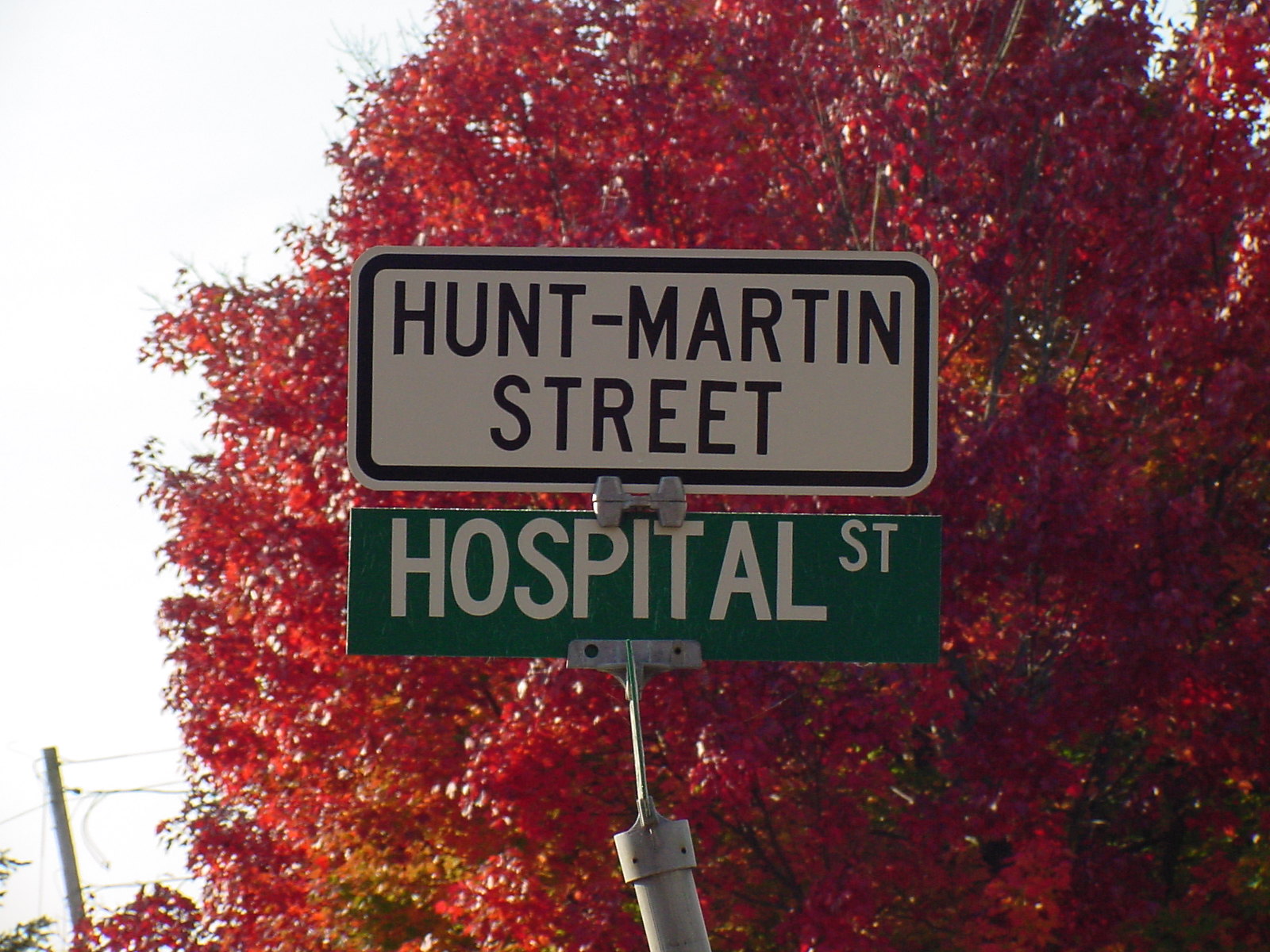The outdoor colour photograph prominently features two North American style street signs mounted one above the other on a single metal pole in the center of the frame. The top sign is a white rectangular sign with rounded corners, outlined by a thinner white and then a thicker black border. The sign reads "HUNT-MARTIN STREET" in bold, black capital letters over two lines. Below it is a narrower green rectangular sign with square corners, also centered on the pole. This sign reads "HOSPITAL" in large white capital letters, followed by "ST" in smaller capital letters towards the top, indicating "HOSPITAL STREET." A dark silver connector partially overlaps each sign. Dominating the background is a vibrant tree adorned with lush, pure red fall foliage, though there are slight hints of green, yellow, and orange towards the bottom of the tree. To the left of the tree is a narrow, slightly curved strip of overexposed sky, appearing almost completely white, and partially visible is what appears to be a telephone pole at the bottom left corner of the image.